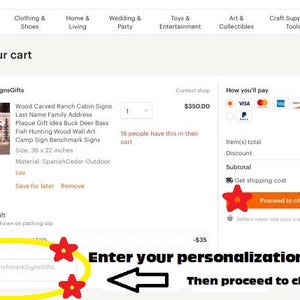The image displays a diverse array of categories and items typically found on an e-commerce website. At the top, there's a navigation bar with categories such as technology, clothing and shoes, home and living, wedding and party, toys and entertainment, art and collectibles, and craft supplies and tools. The gray bar above the categories contains options like "cart" and some unidentifiable text.

In the central part of the image, there's a detailed wooden sign with various themes like cars, ranches, cabins, last names, family entrances, pools, and gift ideas. The wooden sign features intricate designs of bucks, deer, bass, fish, and hunting scenes, and is available in multiple sizes and different types of wood, including Spanish cedar. An option to "save for later" is available. One specific sign costs $350, and it's noted that 60 people have interacted with this item. 

The checkout section shows payment options, including Visa, Discover, American Express, and PayPal. Detailed pricing information is provided, including item total, discounts, and subtotal. A prominent "Get Shopping" button, an orange bar, and a bright yellow circle with red stars are also visible. Additionally, there's a section labeled "Interior Personalization Embassy" with a large arrow pointing to a discount of $35. Some parts of the image appear low quality, making certain details hard to discern.